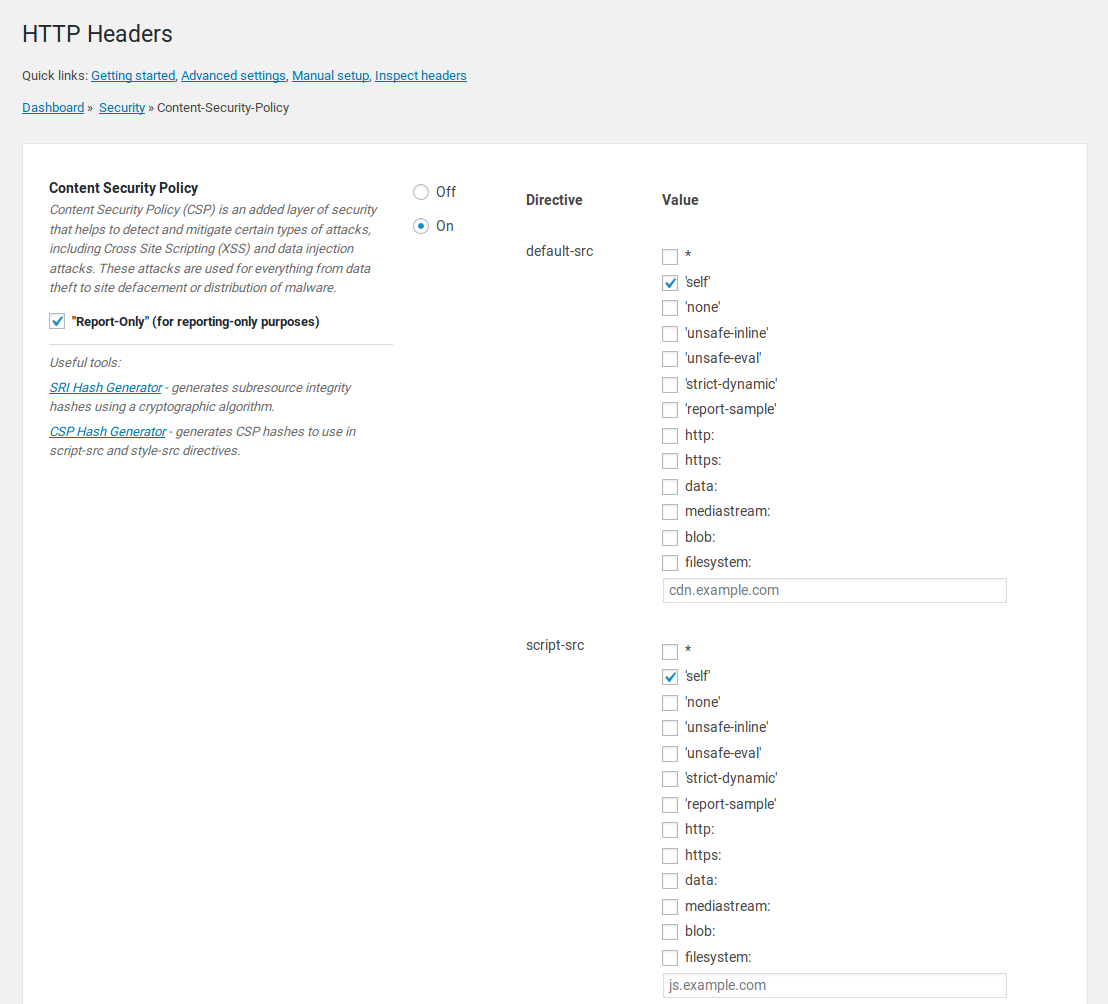The screenshot captures the interface of a website dedicated to managing HTTP headers, with the primary focus on Content Security Policy (CSP) settings.

**Header Section:**
- **HTTP headers**: Main heading.
- **Quick Links**: A menu featuring hyperlinks:
  - Getting Started
  - Advanced Settings
  - Manual Setup
  - Inspect Headers
  - Dashboard
  - Security

**Content Security Policy (selected section):**
- The section is highlighted with a white background and contains the following information:
  - **Definition**: "Content Security Policy (CSP) is an added layer of security that helps to detect and mitigate certain types of attacks, including cross-site scripting (XSS) and data injection attacks. These attacks are used for everything from data theft to site defacement or distribution of malware."
  - **Toggle Switch**: An on/off button with "On" currently selected.
  - **Directive**: Currently set to Default-SRC.
  - **Report Only Option**: A checkbox labeled "Report Only for Reporting Only Purposes" is checked.

**Useful Tools**: Contains hyperlinks and their descriptions:
- **SRI hash generator**: Generates sub-resource integrity hashes using a cryptographic algorithm.
- **CSP hash generator**: Generates CSP hashes to use in Script-SRC and Style-SRC directives.

**Directive Settings**:
- **Default-SRC**: Has multiple value options with checkboxes (most of them are unchecked), including:
  - * (asterisk)
  - self (checked)
  - none
  - Unsafe-Inline
  - Unsafe-Eval
  - Strict-Dynamic
  - Report-Sample
  - HTTP
  - HTTPS
  - Data
  - MediaStream
  - Blob
  - FileSystem

  In this section, there's a specific fill-in-the-blank field with "cdn.example.com".

- **Script-SRC**: Another directive category displaying similar value options, where 'self' is also checked. The fill-in-the-blank field here reads "js.example.com".

**Far Right Column (Value Section)**:
- It includes various values and options mirroring the Default-SRC choices, with a box to check for each. Several options like 'self' and default-src directives are filled in.

This structured and detailed view provides a comprehensive understanding of the website's Content Security Policy management interface, highlighting key settings and options for enhancing web security.